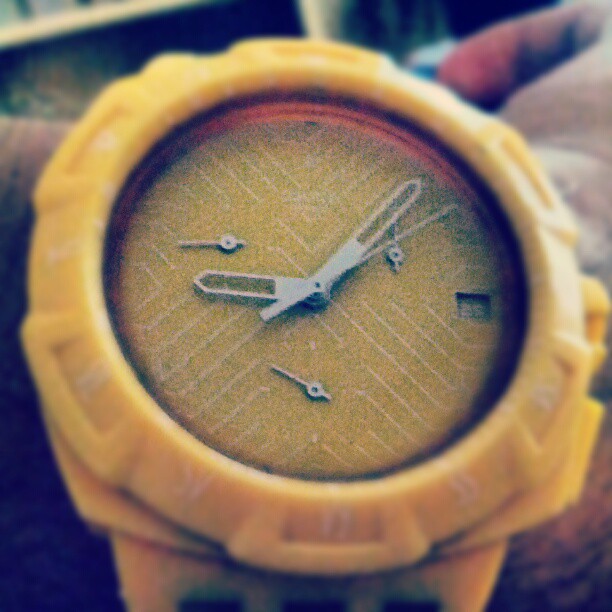A highly detailed close-up photograph of a watch, occupying approximately 95% of the square frame. The watch is worn on a person's wrist and features a striking yellow color theme with a yellow band, yellow face, and yellow trimming around the encasement. The watch face is adorned with silver hands and Roman numerals, though the image is somewhat blurry. Despite the blur, the Roman numerals appear both on the outer casing and on the yellow watch face itself, which is intricately designed with white lines. The timepiece also includes three additional small hands and a square window displaying the date.